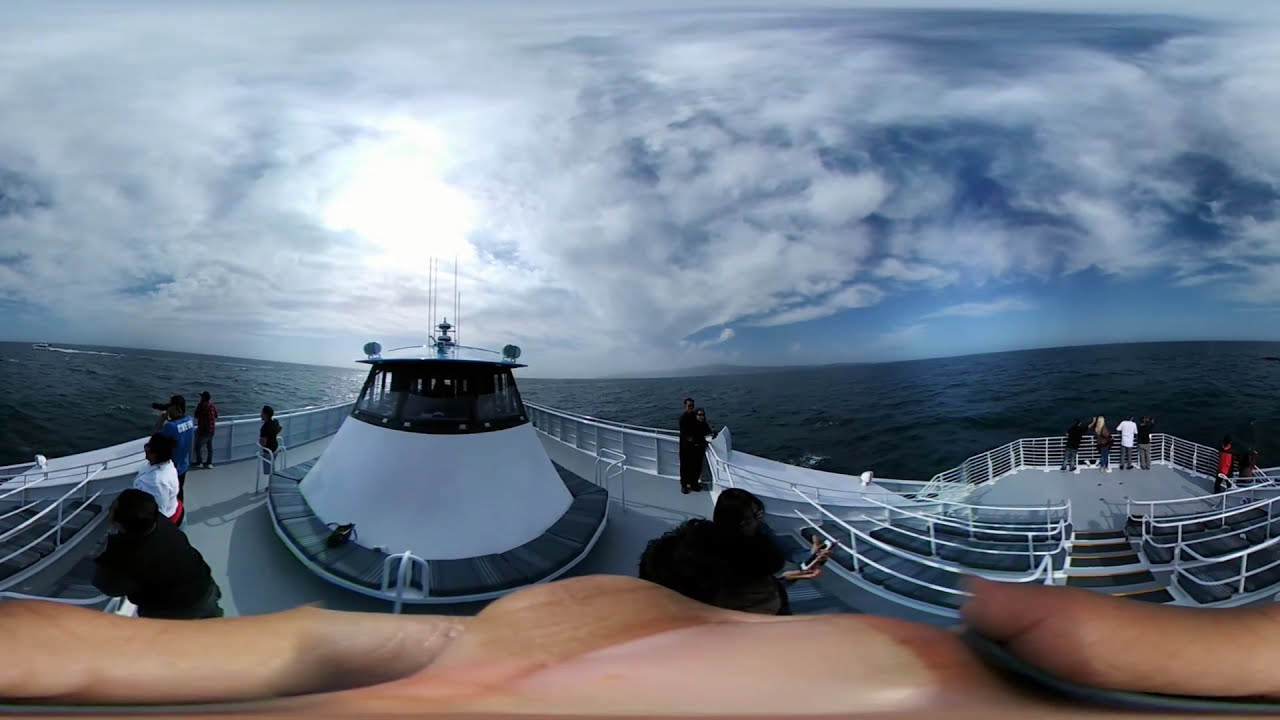This horizontal, rectangular panoramic photograph captures an intriguing scene aboard a white ferry boat. The image, taken with an unusual lens, gives a slightly distorted view, making it challenging to discern the exact orientation of the boat, whether front or back. At the bottom of the frame, the tan fingers of the photographer slightly obstruct the view, adding a candid element. 

Onboard, several people dressed in varied attire—ranging from black to white and blue shirts—stand on the gray deck, clustering around the guardrails and looking outward, possibly whale-watching. The central area of the boat features the cockpit where the captain operates, flanked by empty seating areas. 

Beyond the boat, the dark blue waters stretch out towards a cloudy sky. The sky, predominantly overcast with patches of light blue, suggests possible impending stormy weather. In the distance, a pier and the top of a lighthouse are visible, with the lighthouse's light emitting a glow against the clouds, adding a focal point to the horizon. Overall, the image encapsulates a dynamic maritime scene under a dramatic sky, with elements of human activity, nature, and nautical structures.